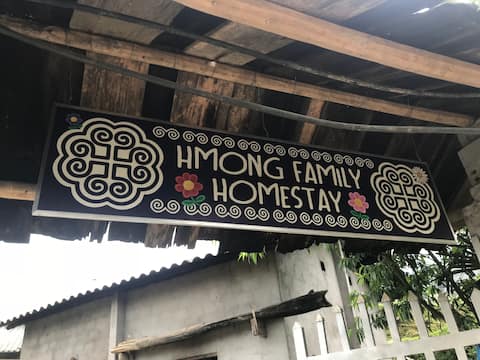The image captures an outdoor scene focused on a large, wooden sign hung from the rafters of a rustic structure, possibly a shed or shack. The sign reads "HMONG FAMILY HOMESTAY" in white capital letters on a black background, with "homestay" positioned below "HMONG FAMILY". Adjacent to the word "homestay" are two flowers: a red-pink flower with a yellow center and green leaves on the left, and a pink flower with a similar yellow center and green leaves on the right. Surrounding the text are curly, swirling graphics that frame the message. The background includes visible wooden rafters, a white fence likely along a walkway leading to the homestay, and a concrete building with a corrugated tin roof. Additional plants and shrubbery are seen behind the fence in the bottom right corner, set against a sky that appears white on the left side, contributing to an overall clear yet detailed portrayal of this homestay sign.